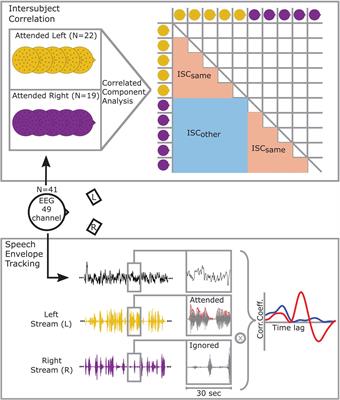The image consists of two detailed graphs stacked vertically. The top graph is titled "Intersubject Correlation." It features a grid with a diagonal line running from the top left to the bottom right. Along the top and side rows of the grid, there are five yellow circles followed by five purple circles, creating a stair-like pattern to the left of the diagonal. Text labels within the graph indicate "ISC same," "ISC other," and "ISC same" once more. Additional notations mention "Attended Left" (N=22), "Attended Right" (N=19), and "Correlated Component Analysis."

Beneath this, the second graph is titled "Speech Envelope Tracking." This section includes various lines in black, yellow, and purple, labeled "left stream" and "right stream." To the right of these primary graphs, there are additional smaller boxes with squiggly lines that feed into a color correlation line. The overall presentation suggests an analysis relating to electrical engineering or signal processing, showcasing intersubject data comparisons and speech signal tracking.